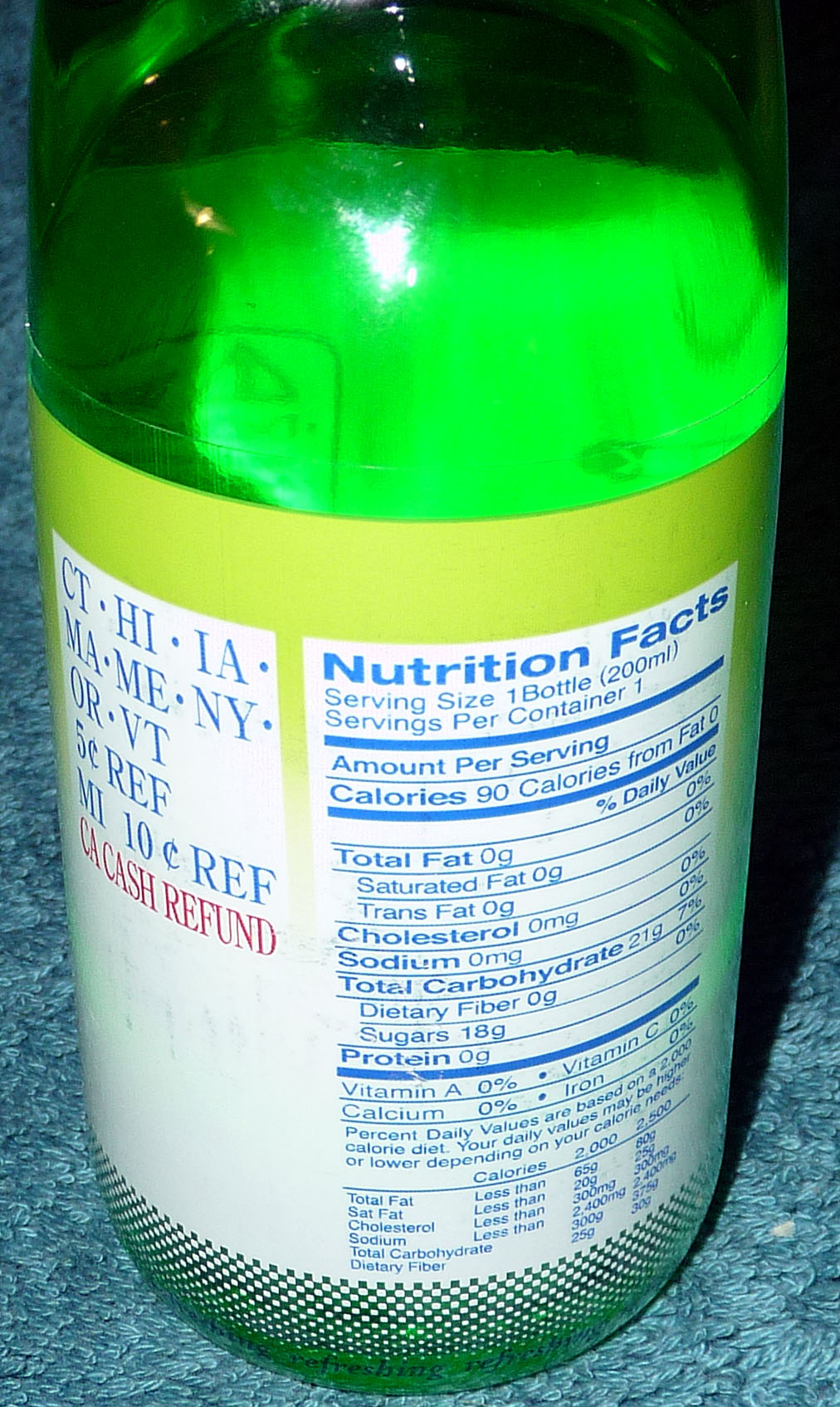A detailed caption for the image could be:

"This image features the back of a green bottle displaying various labels and information. On the left-hand side, there are recycling and refund details, which include 'CT HI IA MA ME NY OR VT 5 cent refund,' 'MI 10 cent refund,' and 'California CA CASH REFUND.' Following these refund details, the label displays 'Nutrition Facts,' outlining dietary information. It specifies a 'Serving Size: 1 Bottle (200 mL),' and indicates 'Servings Per Container: 1.' The nutritional details encompass various components such as total fat, calories, cholesterol, sodium, carbohydrates, among other nutritional elements."